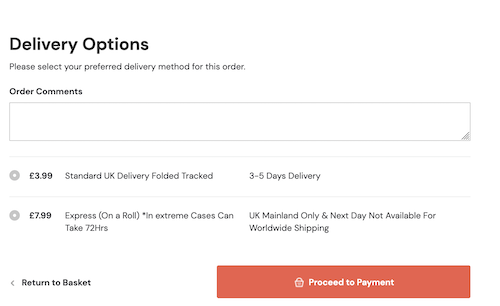The image depicts a webpage focused on delivery options for an order. The background is a bright white, providing a clean and clear interface. All text on the page is in black, with the exception of one red section we'll address later. At the top left of the image, the header "Delivery Options" is prominently displayed in bold black letters. Directly beneath this header, instructional text reads, "Please select your preferred delivery method for this order."

Below these instructions lies a light gray-outlined box labeled "Order Comments." This box has a small corner drag handle in the bottom right for expanding the comment section. Underneath the comment box, the page presents two delivery method options, each represented by a clickable bubble.

The first option is "Standard UK Delivery," which offers folded, tracked delivery within 3-5 days for £3.99. The second option is "Express Delivery," featuring rolled delivery in extreme cases within 72 hours for £7.99. This option specifies it is available only for the UK mainland. It further notes that next-day delivery is not available for worldwide shipping.

At the bottom left corner of the page, there is an option to "Return to Basket." To its right, a prominent red box invites the user to "Proceed to Payment." The overall layout is user-friendly, ensuring clear navigation through the delivery options.